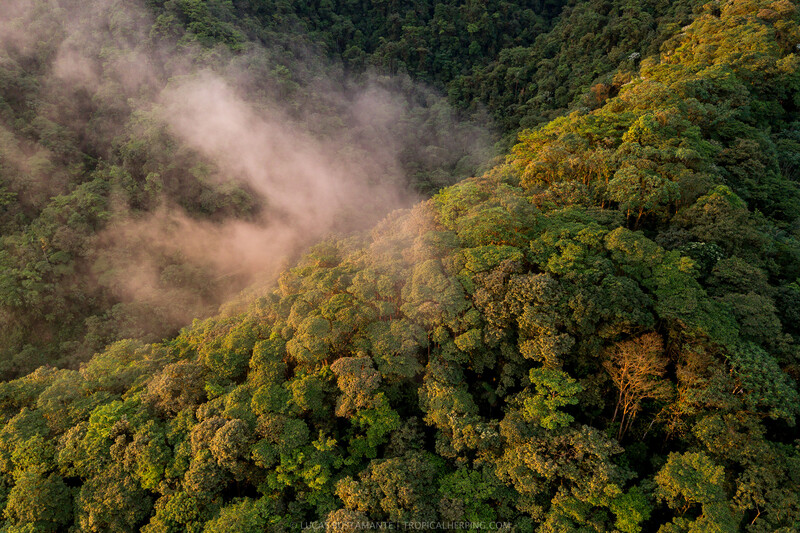This is an aerial view of a densely wooded forest, captured from a high elevation, possibly from a plane. The forest is situated on uneven terrain, giving the appearance of a hill, with the right side ascending uphill and the left side descending into a valley or canyon. The photograph, rectangular in shape, reveals a sea of predominantly green trees interspersed with hints of orange and yellow, possibly suggesting the sun is setting. In the top left corner, there is a large, white, cloud-like formation, which might be a thin layer of clouds or fog, spreading towards the middle of the image. This cloud covers part of a canyon that extends diagonally from the lower left to the upper right, emphasizing the significant elevation difference across the terrain. The intense sunlight and long shadows indicate it is late in the evening. Overall, the image depicts an expansive, vibrant tropical forest with intriguing topographical features and a dramatic interplay of light and shadow.